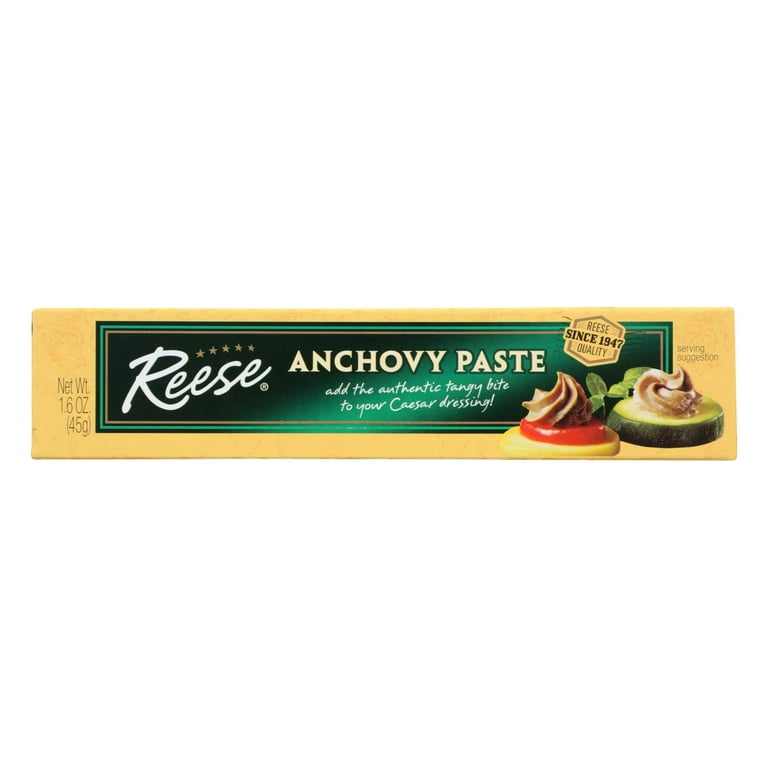The image depicts a rectangular, yellow package of Reese brand anchovy paste, weighing 1.6 ounces (45 grams). The package prominently displays the product name "Reese Anchovy Paste" in bold, brown capital letters. A green label in the middle provides a description: "Add the authentic, tangy bite to your Caesar dressing." Above this, a banner reads "Since 1947 Quality," indicating the brand's long-standing reputation. To the right, there's a serving suggestion showing a cracker topped with anchovy paste and a cucumber similarly garnished, displaying the paste in a decorative swirl pattern. Additional text on the package reads "net weight 1.6 oz or 45 grams," emphasizing the product's lightweight and compact packaging.